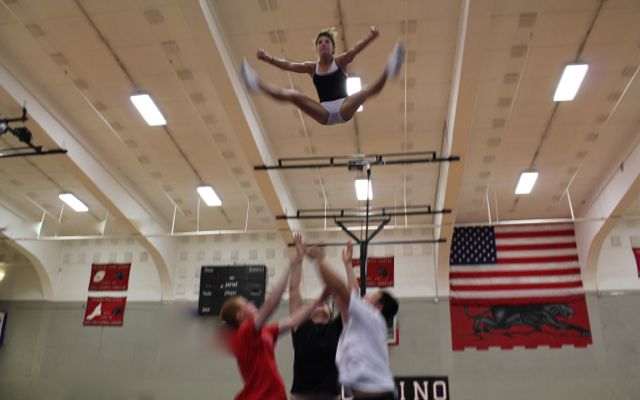The photograph captures the interior of a spacious gymnasium where a gymnastics or cheerleading practice is in session. Dominating the scene is a female gymnast mid-air, jumping with her arms and legs stretched out horizontally to form a V-shape. She is dressed in a black sleeveless top, white shorts, and white shoes. Due to her movement, her feet appear slightly blurry. Beneath her, three individuals—likely men—are positioned to catch her, each with arms fully extended upwards. They are wearing t-shirts in red, black, and white.

The gym's ceiling features rows of fluorescent light fixtures shining down on the scene, creating a well-lit environment. The ceiling and upper sections of the walls are white with gray vent-like squares, while the lower part of the back wall is a darker gray.

In the background, a large American flag is prominently displayed on the right side of the gym wall. Beneath the flag is a red banner depicting a black panther. To the left, there are two vertically-stacked red banners featuring white figures and black text, followed by an inactive black scoreboard. Further left, another set of two similar red banners is visible. The detailed layout suggests a setting rich with school spirit and athletic dedication.